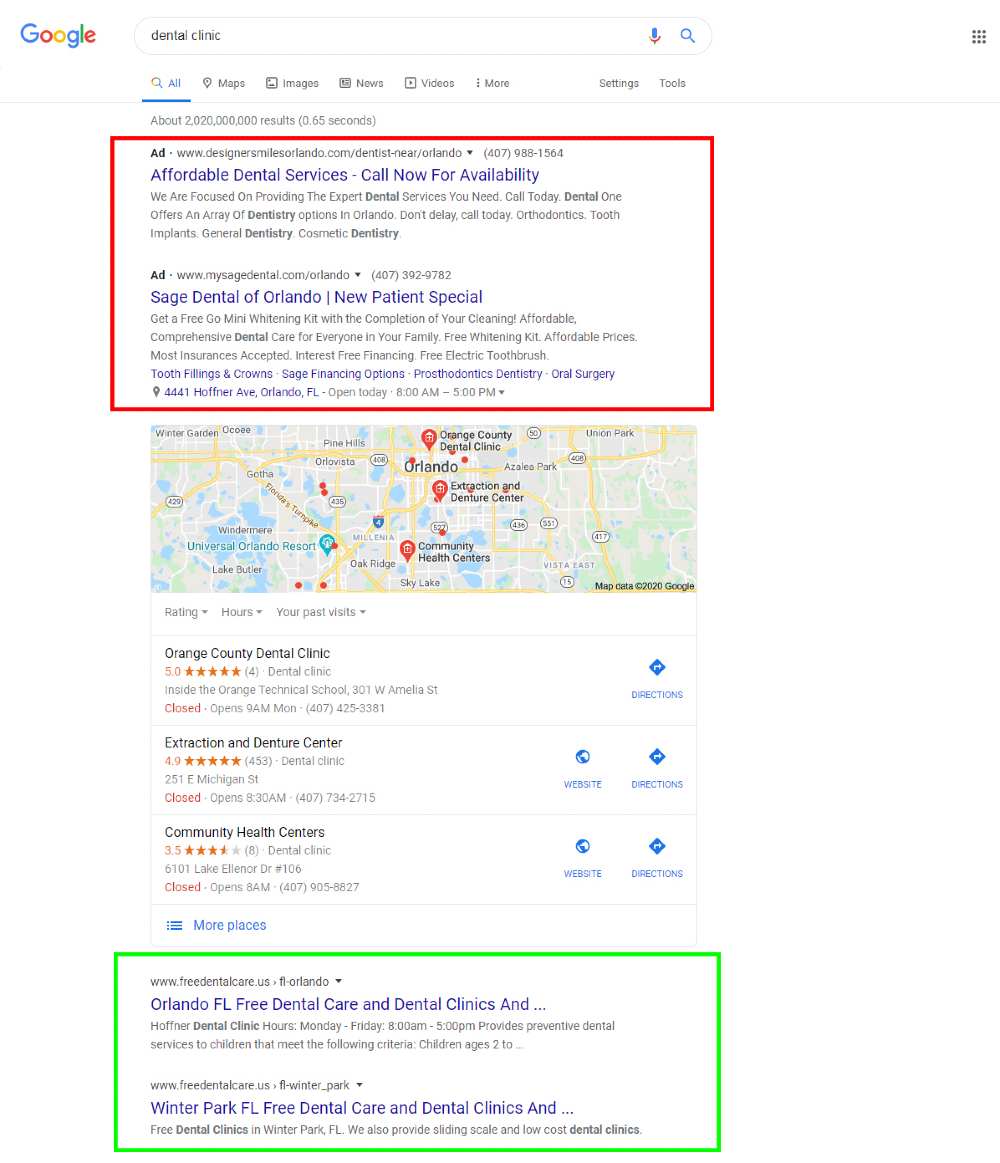The image is a screenshot of Google search results for the query "dental clinic." At the top of the page, it is noted that approximately 2,020,000,000 results were found in 0.65 seconds. Displayed prominently are two ads framed with a red outlined rectangular shape. The first ad is for "Affordable Dental Services," inviting users to call for availability. The second ad is for "Sage Dental of Orlando," highlighting a new patient special. Both ads include descriptions containing their respective website URLs, phone numbers, contact details, and addresses.

Below the ads, Google Maps location search results are shown, featuring a map of Orlando with markers for various dental clinics. The highlighted clinics include Orange County Dental Clinic (5 stars), Extraction and Denture Clinic (4.9 stars), and Community Health Centers (3.5 stars).

Further down, encased in a green rectangle, are two non-sponsored results. The first one is titled "Orlando FL Free Dental Care and Dental Clinics," with an ellipsis indicating more text follows. The second is titled "Winter Park FL Free Dental Care and Dental Clinics," also followed by an ellipsis.